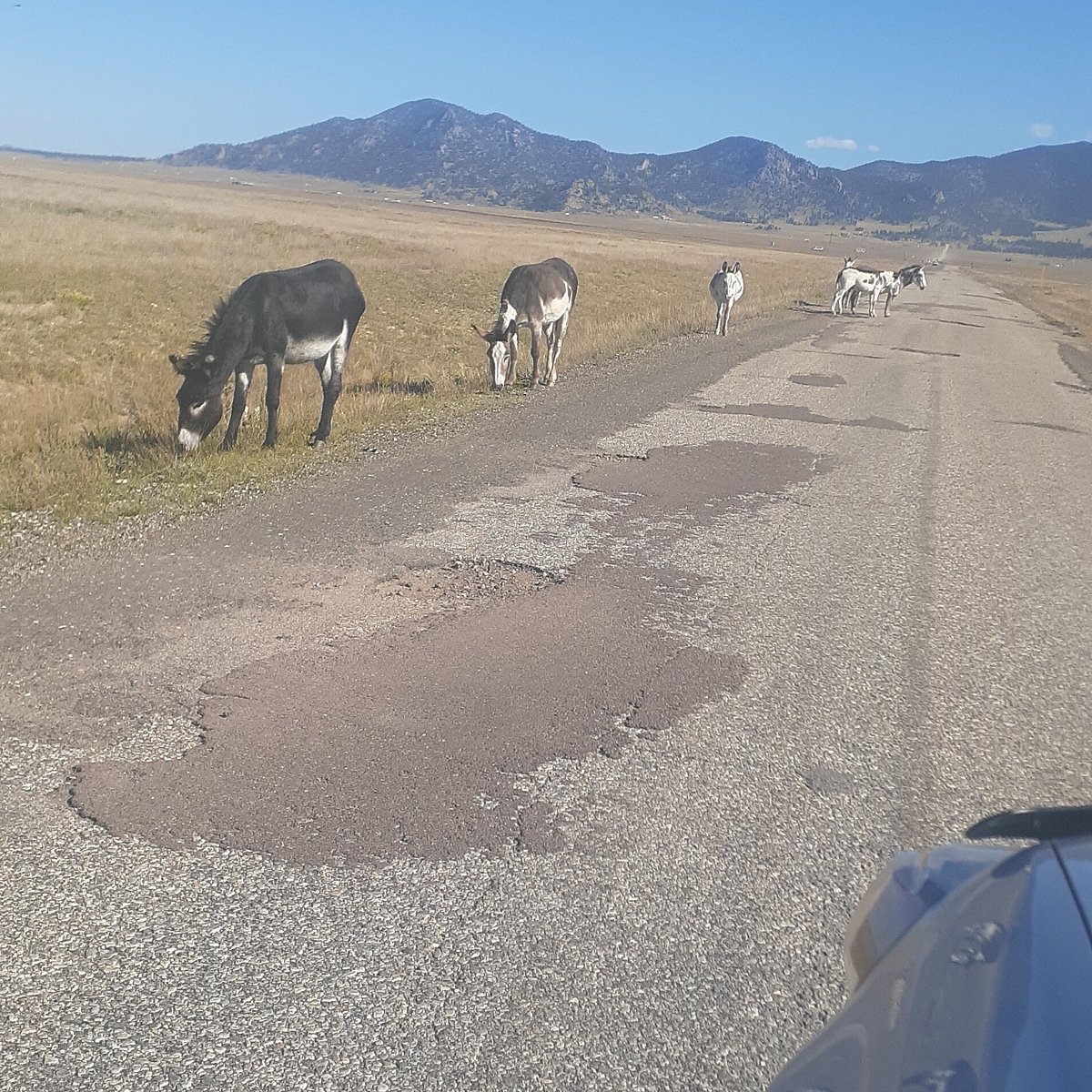This poorly-focused photograph, likely taken with a phone from the window of a car, captures a charming countryside scene. It features a group of five donkeys grazing along a patchy, mostly unpaved road that stretches diagonally from the lower left to the top right of the image. The road, showing signs of age with faded lines and pothole repairs, winds through a serene landscape of light green and yellow grass, which appears lush near the road but gradually turns brown toward the background. In the distance, a range of mountains rises under a bright blue sky dotted with a few clouds. The donkeys, either standing or feeding on the grass, add a whimsical touch to this quaint outdoor setting, further enhanced by the presence of a car's corner in the bottom right, hinting at the spontaneous nature of this snapshot.